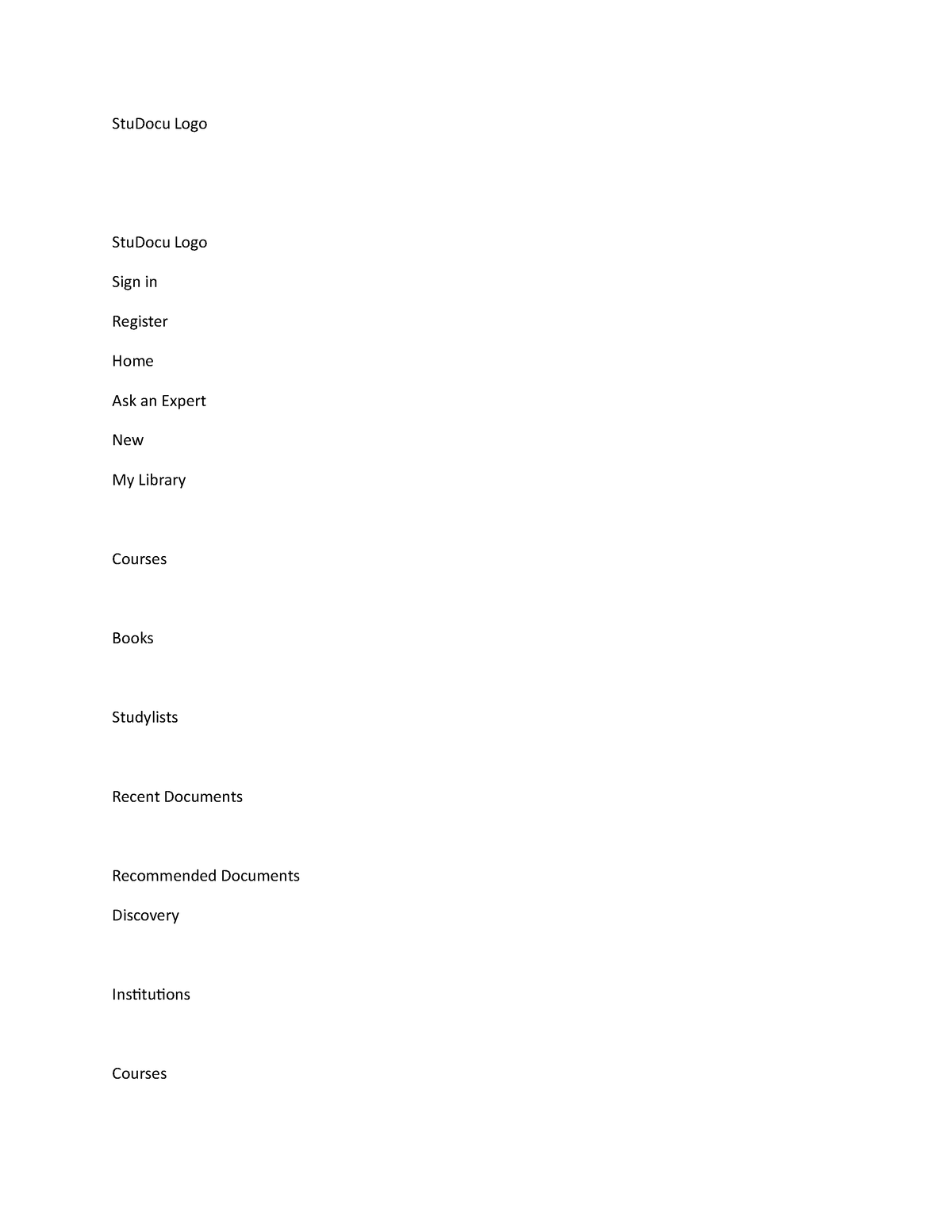The image is a screenshot of an application interface featuring various sections. At the top, the header displays the "stu.co" logo alongside navigation options: "Sign In" and "Register." The main menu items, listed on the left side in a left-aligned format against a white background, include: "Home," "Ask an Expert," "New," "My Library," "Courses," "Books," "Study Lists," "Recent Documents," "Recommended Documents," "Discovery," "Institutions," and "Courses." Each section is clearly delineated, providing a comprehensive overview of the app's extensive resources and features.